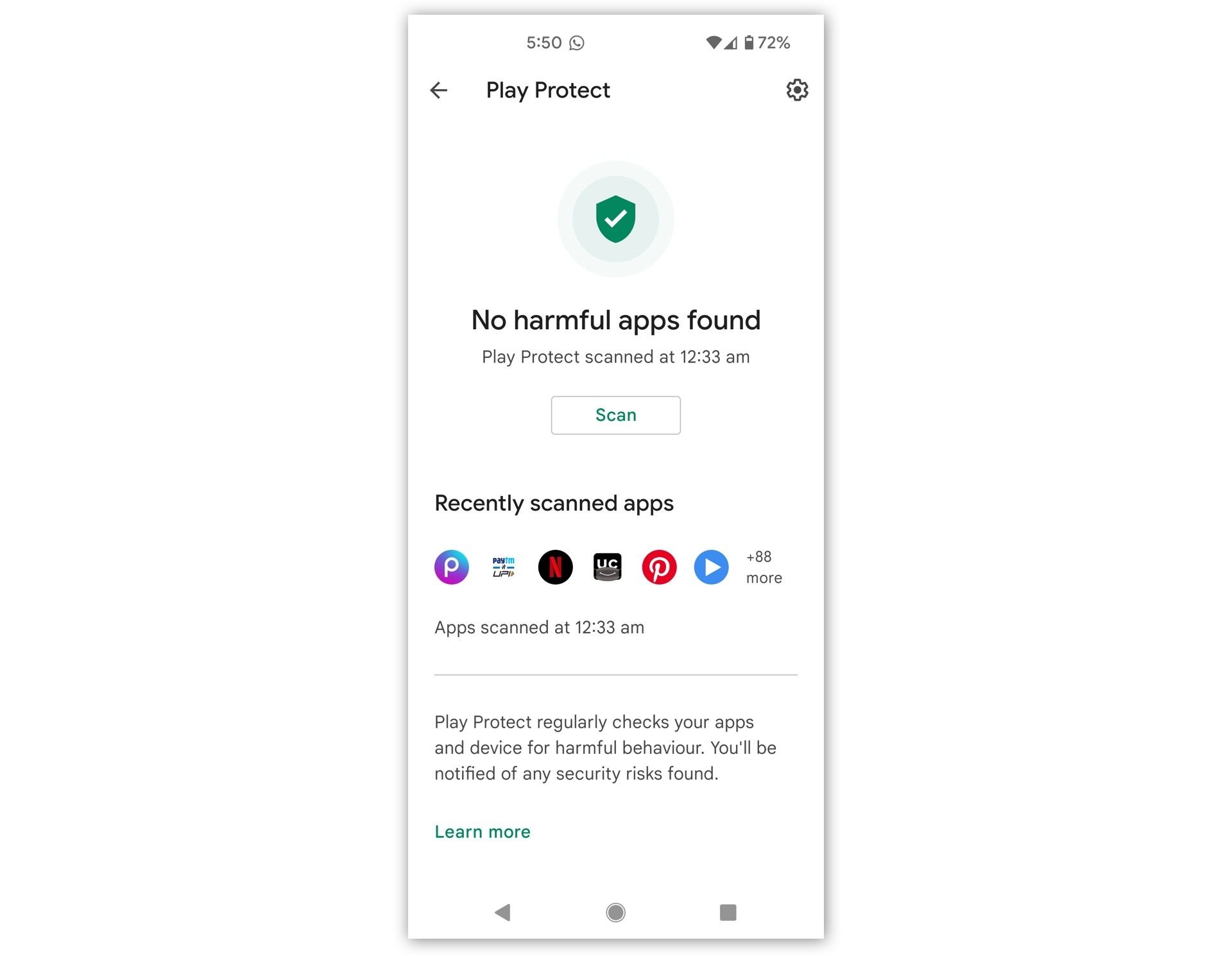Screenshot of an Android phone displaying a Play Protect scan result. The top section shows standard Android elements including signal strength, Wi-Fi, battery status, and the time against a white background. Below these indicators, the title "Play Protect" is flanked by a back button on the left and a settings gear icon on the right. A prominent green shield icon with a checkmark is displayed, accompanied by the message "No Harmful Apps Found." The scan was completed at 12:33 a.m., suggesting the image is related to mobile security.

Following this, a green "Scan" button is enclosed in a grayish-lined rectangle. Directly below, the text "Recently Scanned Apps" appears above a row of app icons including Netflix and Pinterest, among others, with "Plus 88 More" noted to the right, indicating additional apps were scanned at the same time.

The message "Play Protect regularly checks your apps and device for harmful behavior. You’ll be notified of any security risks found" is displayed beneath the scanned app details. A "Learn More" link in green font suggests additional information is available. Finally, at the bottom of the screen are playback control buttons: a reverse button on the left, a circular record button in the center, and a stop button represented by a gray square on the right.